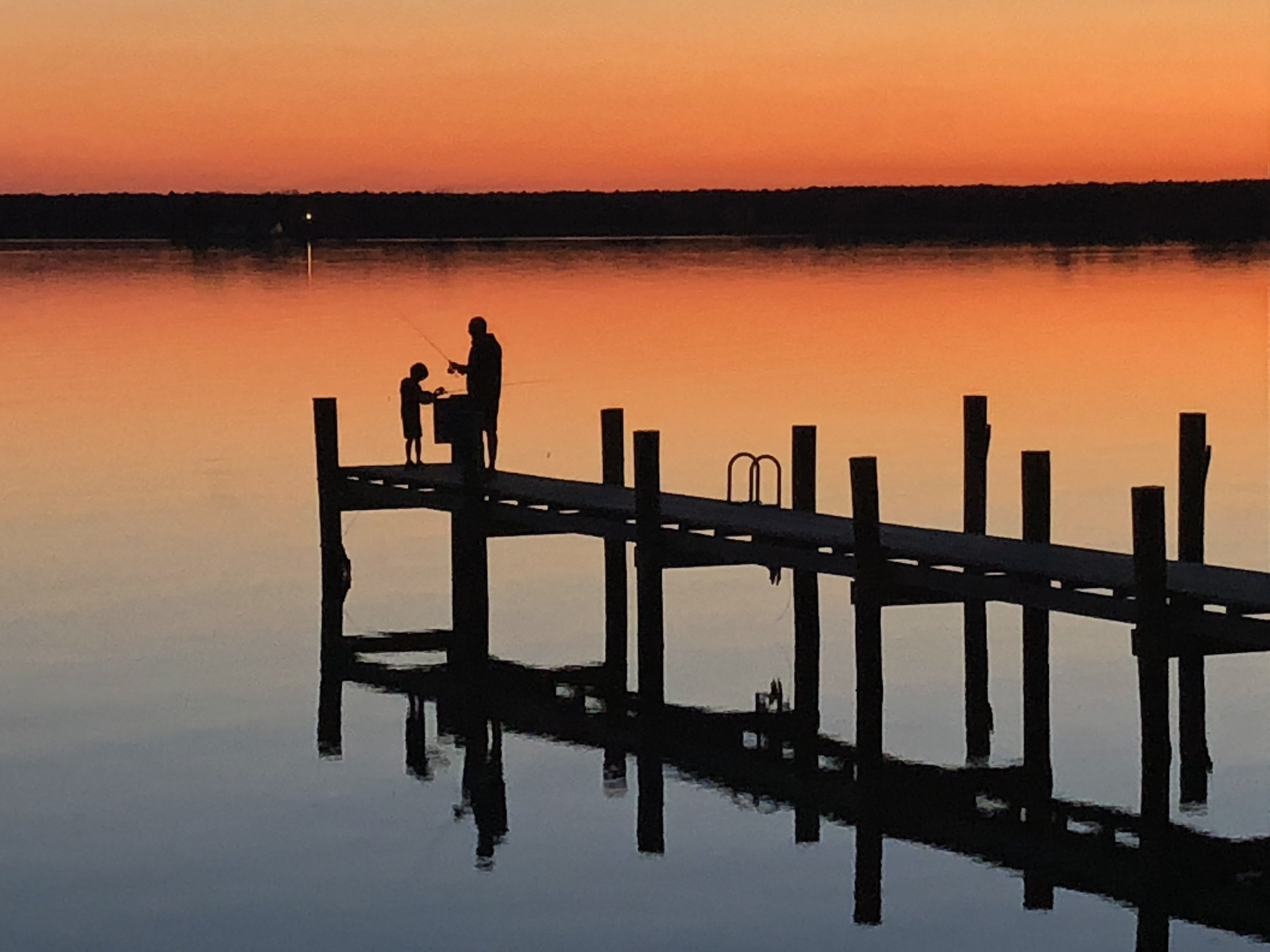The photograph captures the serene moment of an elderly man and a young boy, likely his grandson, fishing off a wooden pier that extends from the bottom right corner towards the center left of the image. Both figures are silhouetted, but it's clear they are holding fishing rods and reaching into a cooler, possibly for bait or packing up for the day. The backdrop features a breathtaking sunrise or sunset, with a gradient of vibrant oranges and yellows merging into the tranquil blue of the lake's water. The horizon is notably straight, with a dark, flat landscape marked by a thin black line of trees, and distant lights hinting at the presence of a house, boat, or car. The pier, though appearing unstable with its hastily constructed look and protruding support poles, casts a mirror image onto the calm water, enhancing the peaceful yet poignant atmosphere of two generations bonding by the water's edge.